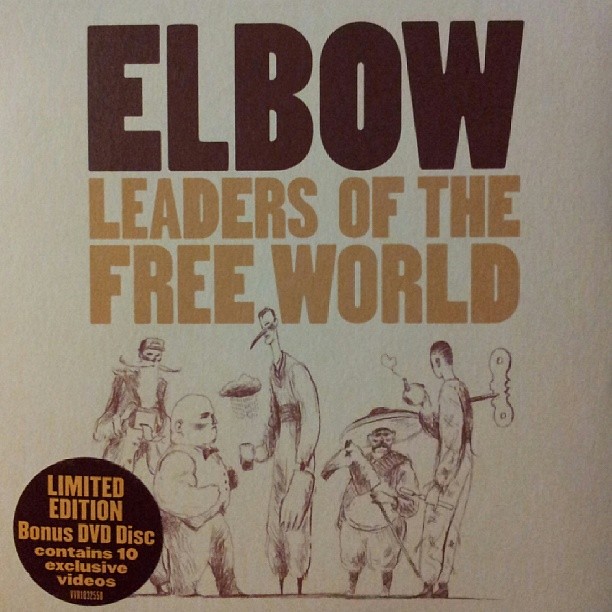This is the cover of a Limited Edition Bonus DVD for "Elbow: Leaders of the Free World." The cover has a textured cardstock appearance and is predominantly gray with a white top section. At the top, the title is prominently displayed with "ELBO" in large, dark brown letters and "Leaders of the Free World" in slightly smaller, light brown letters. Beneath the title, the cover features a detailed illustration of five cartoon characters. On the far left, there is a man with a handlebar mustache and long beard, holding a box. Next to him is a short, stout man wearing a black bow tie and vest. The central figure is the tallest, an extremely skinny man with a long pointy nose, holding a glass of what appears to be a dark drink. To his right is a man wearing a large sombrero, depicted in a stereotypical Mexican style, holding a toy horse stick. The figure on the far right has a wind-up crank protruding from his back and is holding a large tool. In the lower left-hand corner, there is a dark brown circle with goldish beige text that reads "Limited Edition Bonus DVD Disc Contains 10 Exclusive Videos."